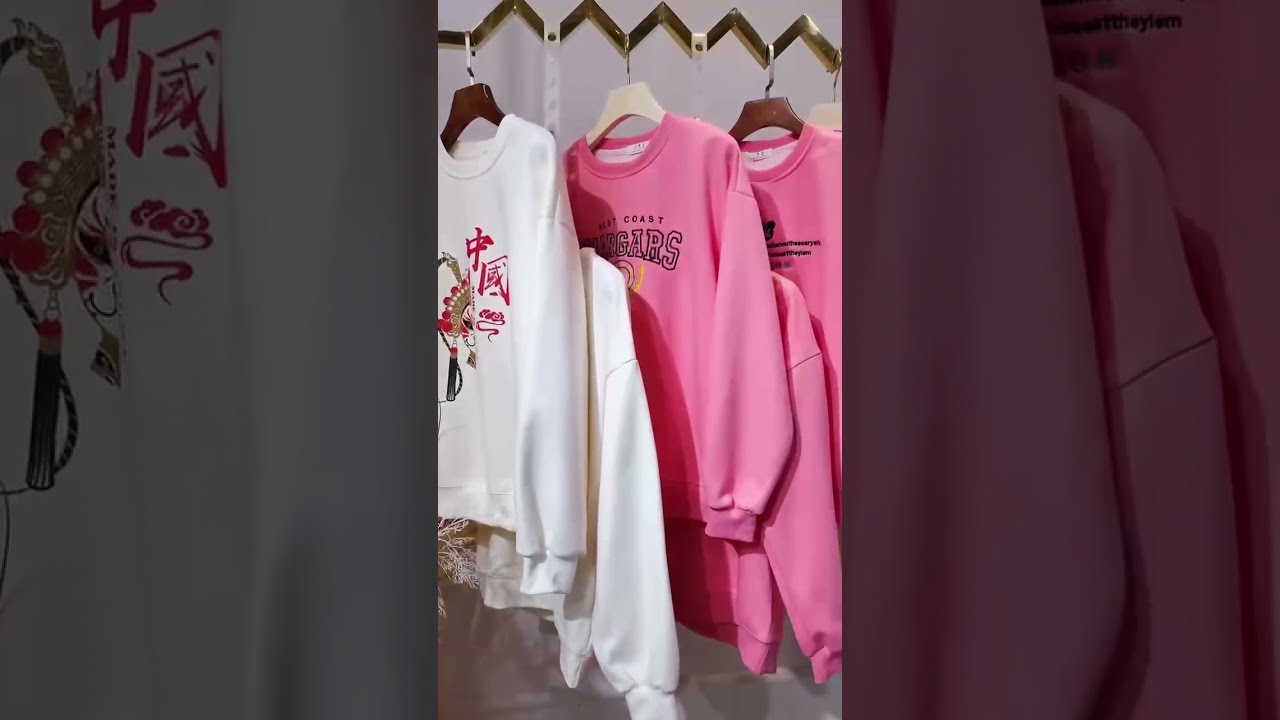The image depicts an arrangement of sweatshirts hanging from a goldish, zigzagging pole in what appears to be a closet. On the left, a brown wooden coat hanger displays a white sweatshirt adorned with a dragon design and Asian characters. Another white sweatshirt, hanging slightly lower, is supported by a white strap rather than a hanger. In the center, a pink sweatshirt on a white hanger has partially visible text that seems to spell "West Coast Jaguars." Behind it, another pink sweatshirt hangs from a strap, followed by an additional pink sweatshirt on a wooden hanger. The image composition emphasizes the alternating pattern of the sweatshirts, creating a staggered effect that reveals parts of the garments while obscuring others. The setup seems characteristic of a social media post, possibly a TikTok screenshot, highlighting the organization of the sweatshirts in a visually engaging manner. A vertical view suggests that the image captures the top clothes-hanging area of the closet, framed by a blown-up background that enhances the overall aesthetic.